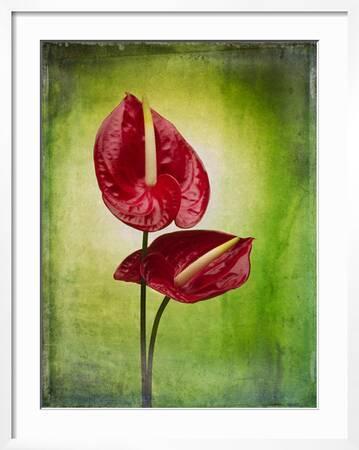This lower-quality photograph captures an intricately framed artwork, featuring a striking depiction of two red calla lilies with prominent thick white or yellowish stamens at their centers. The flowers are set against a grungy green backdrop that transitions from bright green in the center to darker hues at the edges, accentuating the vibrant red petals. The taller flower stands prominently while its companion curves gracefully downward to the right. The artwork, although its medium remains ambiguous between a painterly photograph and a realistic painting, is mounted in a white matte within a white picture frame. The background transitions from a yellow-white behind the flowers to varying shades of green, adding depth and contrast to the image. The image contains no visible signatures, people, animals, structures, or machinery.